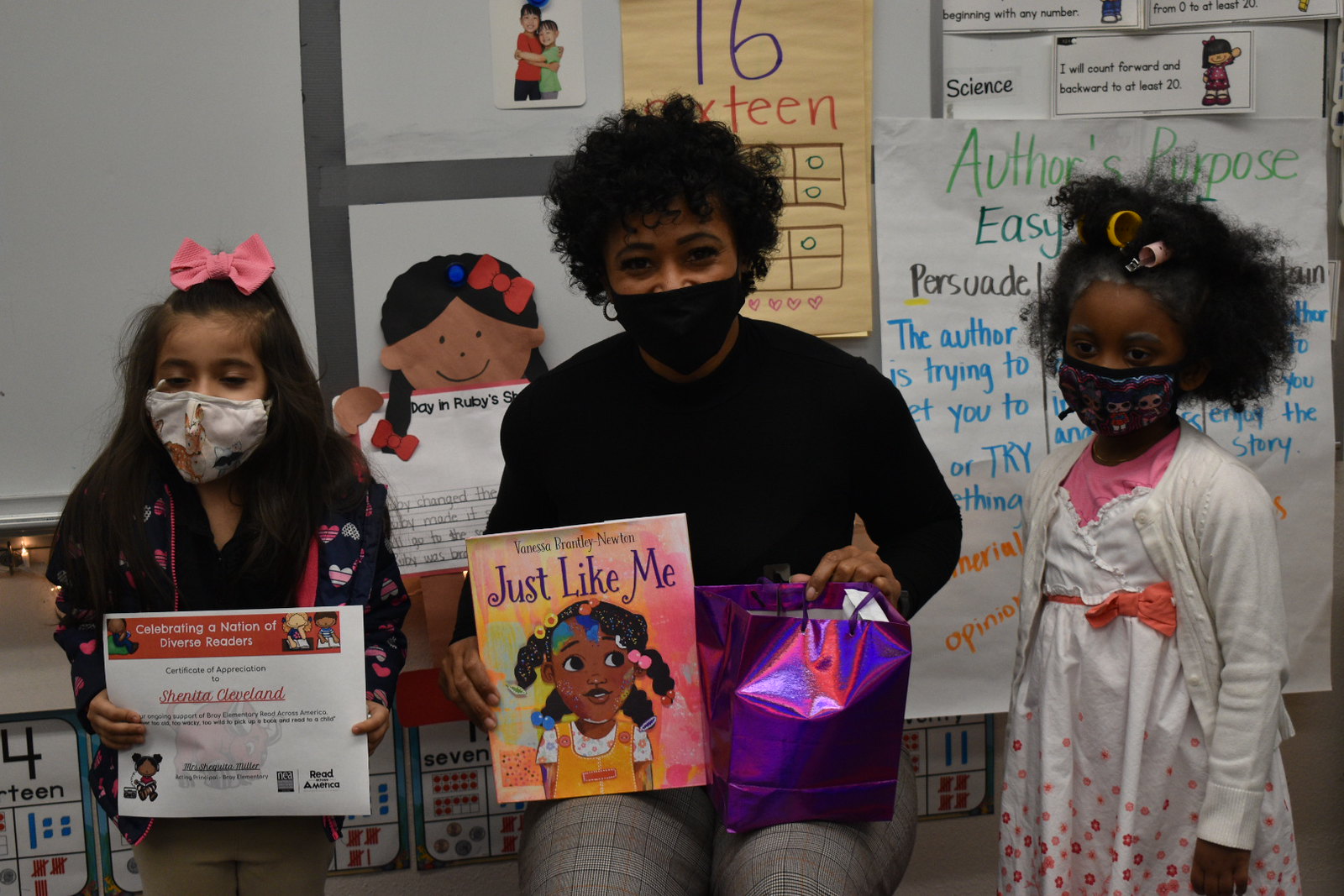In a lively elementary classroom adorned with educational posters and stickers, an African American woman, presumably the teacher, stands at the forefront, holding a book titled "Just Like Me" featuring a watercolor illustration of a young Black girl. She also clutches a purple gift bag. The teacher, with her short curly hair and a visible smile through her face mask, is flanked by two children. On her right stands an African American girl in a white dress with a pink undershirt and a red sash or tie. On her left, a younger Hispanic girl, wearing a black outfit decorated with colorful hearts and a pink bow in her hair, holds a "Celebrating a Nation of Diverse Readers" certificate with her name, Shanita Cleveland, written on it. Despite the vibrant classroom setting and the teacher's enthusiastic demeanor, the two children appear tired and somewhat ready for the moment to end.